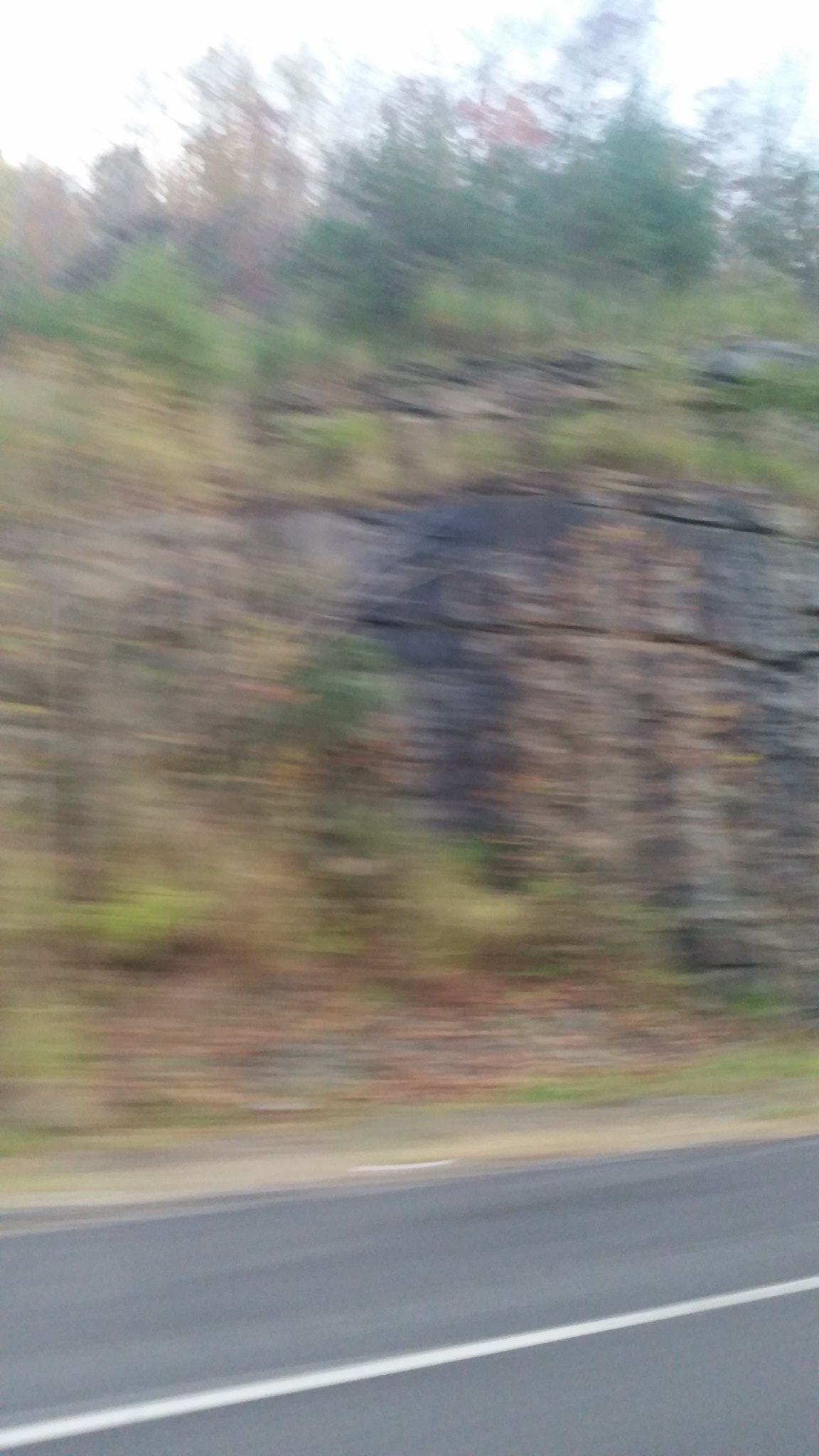This dynamic photo, likely shot from a swiftly moving vehicle, captures a striking vertical perspective of a roadside landscape. The image's foreground features a blacktop road divided by a singular long white solid line marking the center between two lanes. Adjacent to the road lies a stretch of gravel interspersed with patches of brown and green scrub brush. The scene progresses into a sharply cut rock face, suggesting the deliberate work of heavy machinery due to its remarkably flat surface. The rock is primarily dark gray, streaked with intermittent layers of tan. Rising above the rock face, more scrub brush and rocky outcrops can be seen, eventually giving way to a dense cluster of trees comprising both fir and deciduous varieties. The backdrop is dominated by a dazzlingly bright, white sky, adding a dramatic contrast to the rugged terrain below.